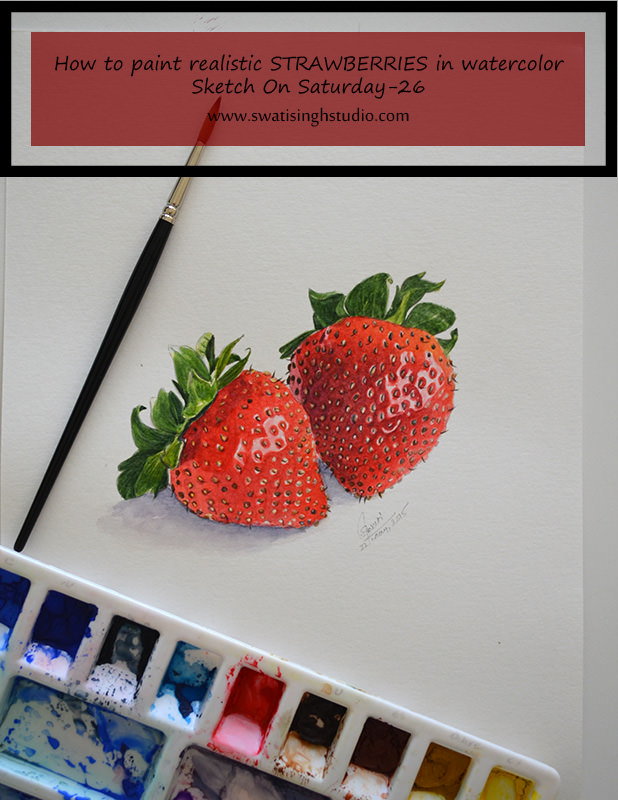The image portrays a sophisticated advertisement for a painting class, teaching "How to Paint Realistic Strawberries in Watercolor" as part of the series "Sketch on Saturday - 26." The advertisement, which could be a leaflet or digital, prominently features black text against a translucent red backdrop at the top, with the web address, www.swattenbergstudio.com.

Central to the visual composition are two meticulously painted red strawberries, complete with delicate seeds and vibrant green leaves, capturing light and shadow exquisitely for a realistic effect. The strawberries are situated on a white background, highlighted by expert shading that brings out the texture and form. A paintbrush lies beside the strawberries, suggesting the tools used, and below them, a well-used palette resembling a white plastic ice cube tray is filled with various splattered colors of watercolor paints. The image is rectangular with vertical sides being longer, and the overall artistry provides a compelling invitation to the painting class.